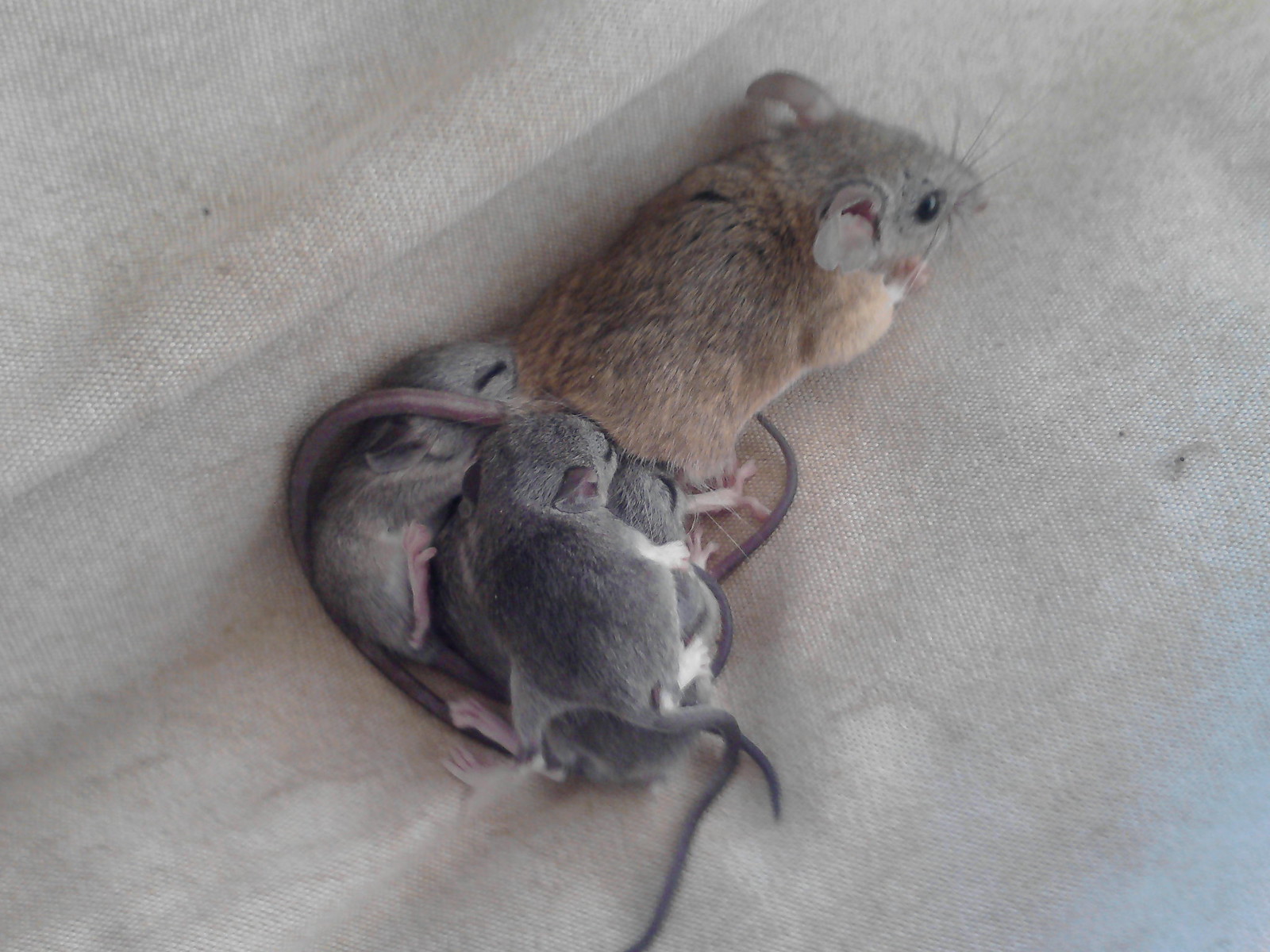This image showcases a charming scene of a light brown field mouse with three tiny, adorable baby mice nestled closely behind her. The mother mouse, distinguishable by her grayish face, open eyes, and tender whiskers, is perched on an off-white, cream-colored piece of fabric. The baby mice, with their delicate gray bodies, pink feet, and long tails, are endearingly piled up on one another as though they are seeking warmth and comfort near their mother's bottom. With their eyes still shut, indicating their very young age, the little ones appear to be nursing or attempting to snuggle underneath their mother. The soft folds of the fabric suggest the setting might be a cozy, indoor environment, possibly hinting that this could be someone’s beloved pets. The scene exudes a tender and heartwarming vibe, capturing the softness and cuteness of a mouse family in a serene, nurturing moment.